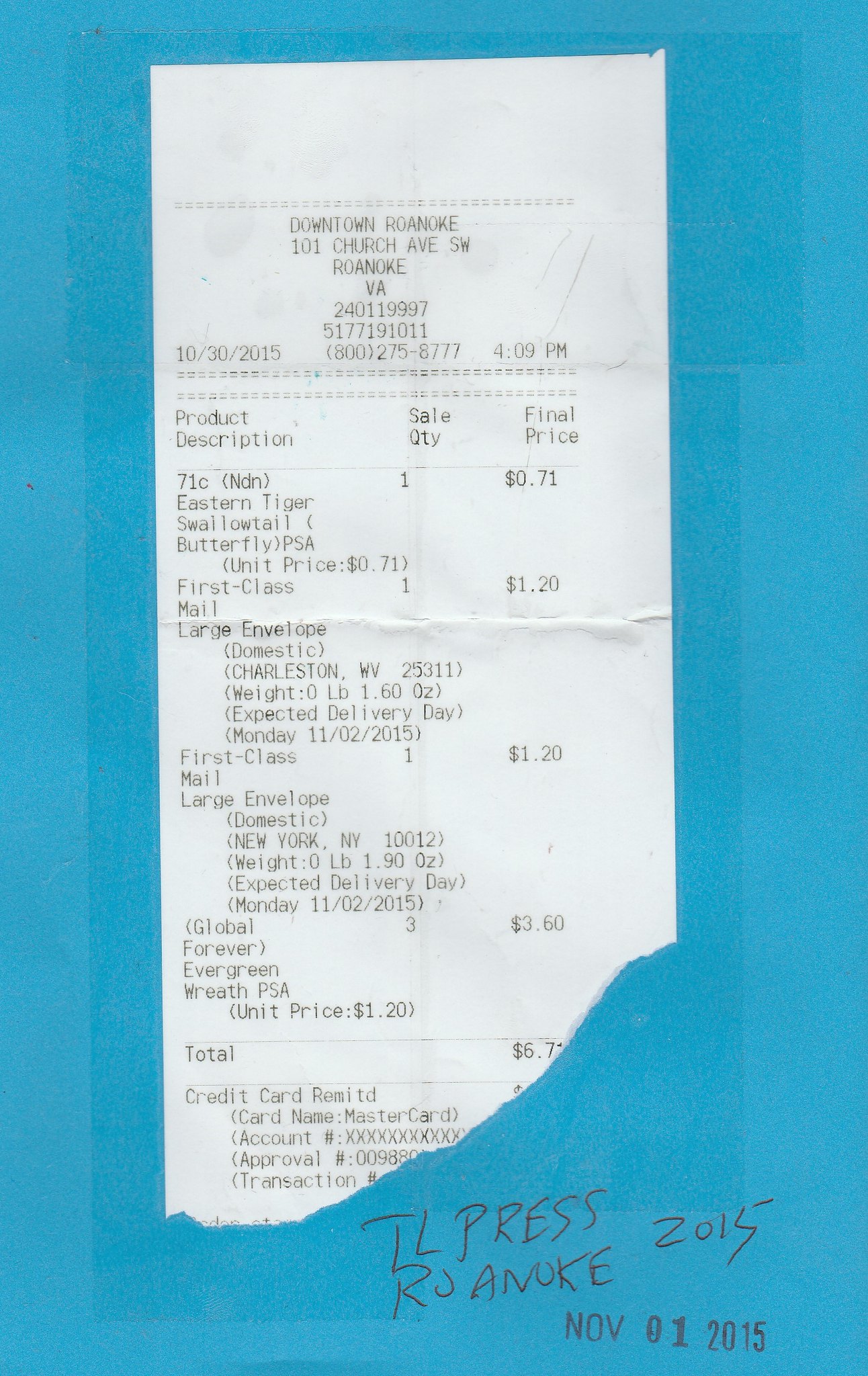The image features a tall, vertically-oriented rectangle that's approximately two and a half times taller than it is wide, set against a light teal background. This background contains creases that form a vertical rectangle occupying the majority of the bottom two-thirds of the image, with another slightly wider horizontal rectangle intersecting it.

Prominently displayed in the center from top to bottom is a black-and-white receipt. The receipt's text is small, but several details are discernible. It is from "Downtown Roanoke," specifically at "101 Church Street Ave. Southwest, Roanoke, Virginia." Besides the location, the receipt includes various numbers, such as the date, which appears to be "November 01, 2015," along with a phone number.

The content of the receipt indicates the purchase of an "Eastern Tiger Swallowtail Butterfly," classified as first-class mail. There are also mentions of large envelopes and a wreath. The total price of the purchase is listed as $6.70, although the receipt appears to be torn at the bottom right, slightly obscuring the last digit. Additional text at the bottom right of the image reads "TLPRESS ROANOKE 2015" along with "01 2015."

Overall, the image is a visually detailed scene, primarily focused on the intricacies and specifics of the receipt set against a uniquely creased teal backdrop.